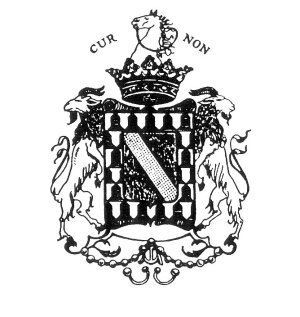The image is a black and white hand-drawn crest, designed in a classic royal style. It's a small depiction set against a white background. At the very top of the crest, there is a detailed drawing of a horse's head, outlined in black and facing to the left. Flanking the horse's head are the letters "C-U-R" on the left and "N-O-N" on the right, in bold black lettering. Directly below the horse's head sits a crown, also intricately outlined in black.

The main body of the crest features two lion-like figures with goat heads positioned on either side, each seeming to balance on the edges of a shield-like object. These goat-headed creatures are depicted with a sense of motion, each looking away from the center crest. The central shield-like portion of the crest has a distinct checkered pattern with alternating black and white squares, lending the emblem a sense of texture and depth. The outer edges of this central shape are adorned with white, bullet-like shapes.

Below the main body of the crest, there's a decorative element resembling beadwork or a beaded necklace with two small looped piercings hanging below it, adding a finishing touch to this intricate and elaborate design.